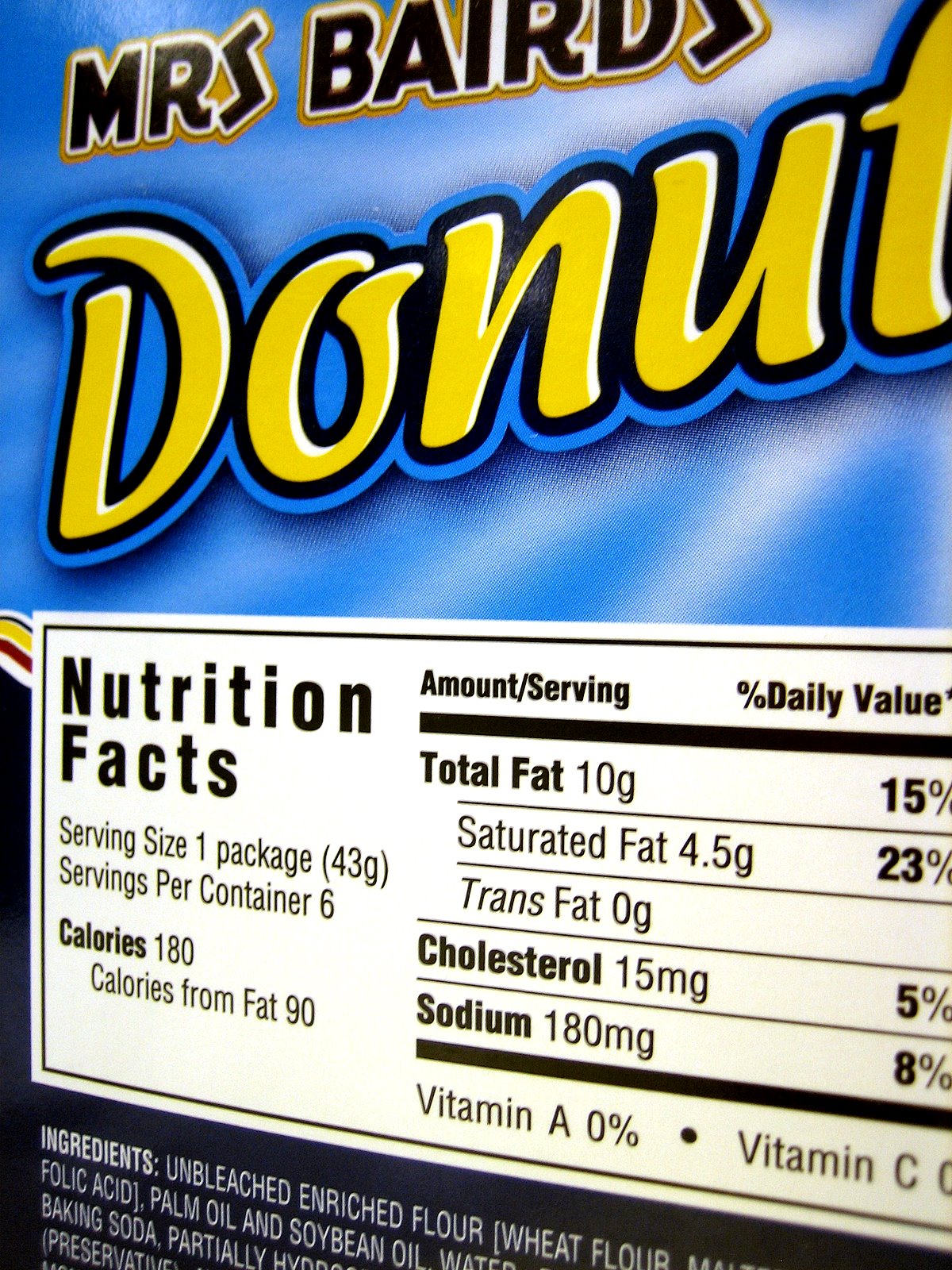This image features a close-up shot of a box of donuts branded "Ms. Bard's Donuts." The packaging predominantly uses light blue and white colors, with darker blue shading along the bottom edge. At the top of the box, "Ms. Bard's Donuts" is prominently displayed. Below this, a small rectangular white table provides nutritional information, listing details such as total fat, saturated fat, trans fat, cholesterol, sodium, vitamin A, and vitamin C. It indicates that the package contains six servings. Also, the calories per serving and various ingredients are detailed at the bottom of the box. The image zooms in closely on the packaging, emphasizing these informative elements.